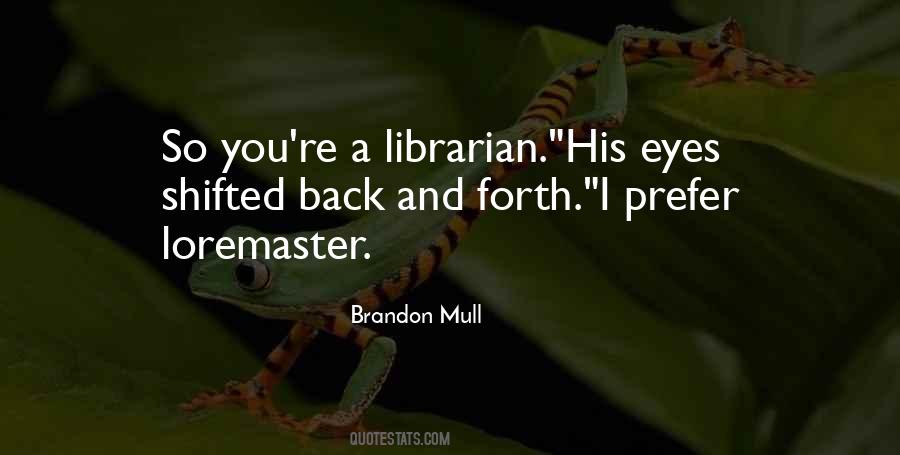This poster features a white text quote that reads, "So you're a librarian? His eyes shifted back and forth. I prefer Loremaster." Beneath it, the author's name, Brandon Mull, is displayed alongside the source, quotestats.com. The background image features a vivid green frog with an orange and black-striped underbelly, captured mid-jump between two green leaves. Despite the frog's striking colors, the image is darkened to emphasize the text, making the words the focal point. The overall poster, which is twice as wide as it is high, combines the darkened photograph with a black and green color scheme that complements the frog and the foliage.